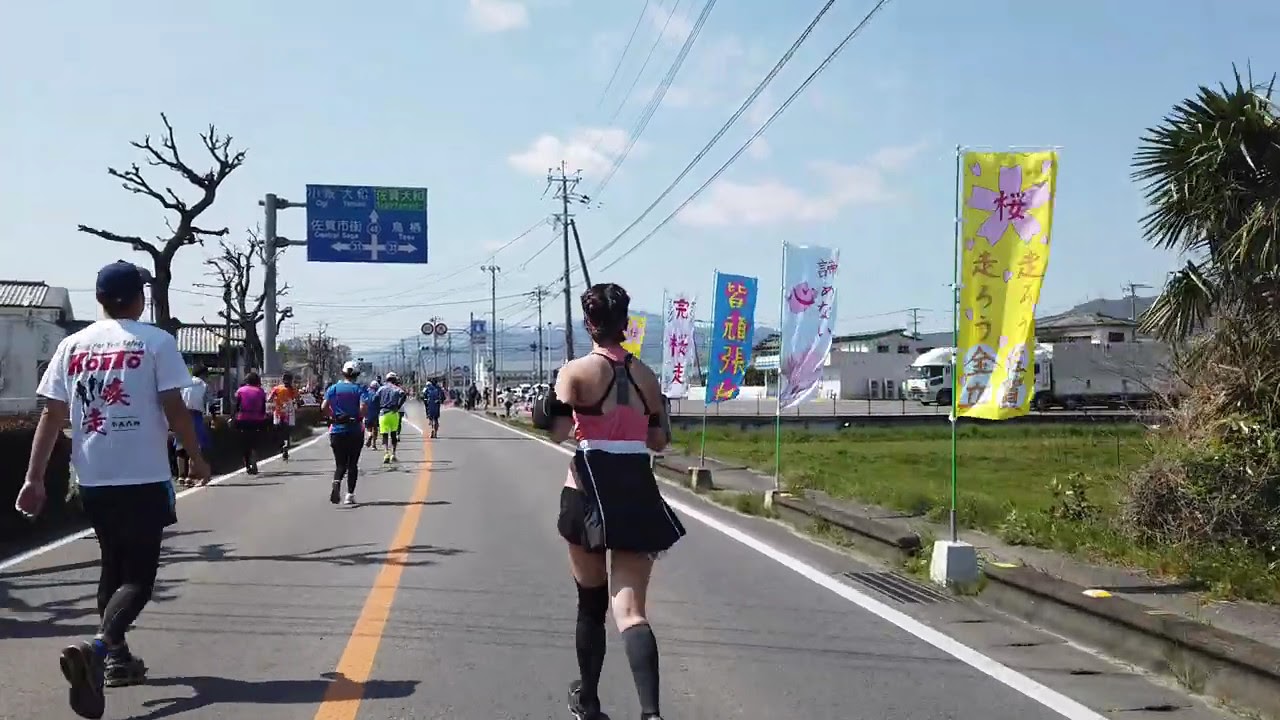The photograph captures a vibrant road race likely taking place in Japan. Dominating the center of the image is a paved street with a distinct yellow line down the middle and white lines marking the edges, which separate the road from the grass and a small curb on the right side. The sky overhead is blue with few clouds, allowing for a bright and clear daytime setting. In the foreground, a woman dressed in a pink blouse, black skirt, and black socks, is running, while to her left is a man wearing a white and red T-shirt, dark shorts, and dark socks. Several other participants are visible further ahead, jogging or walking. Along the right side of the road are numerous banners on thin green poles, with bright yellow, white, and blue backgrounds, all bearing Japanese characters. The roadside also features a shrub, and further beyond, some buildings and trucks can be seen. Overhead, telephone lines stretch across the scene. On the left side of the road, a barren tree and a large blue street sign on a gray pole are noticeable, suggesting directions to various destinations. The overall atmosphere of the image conveys the energetic spirit of a community marathon.